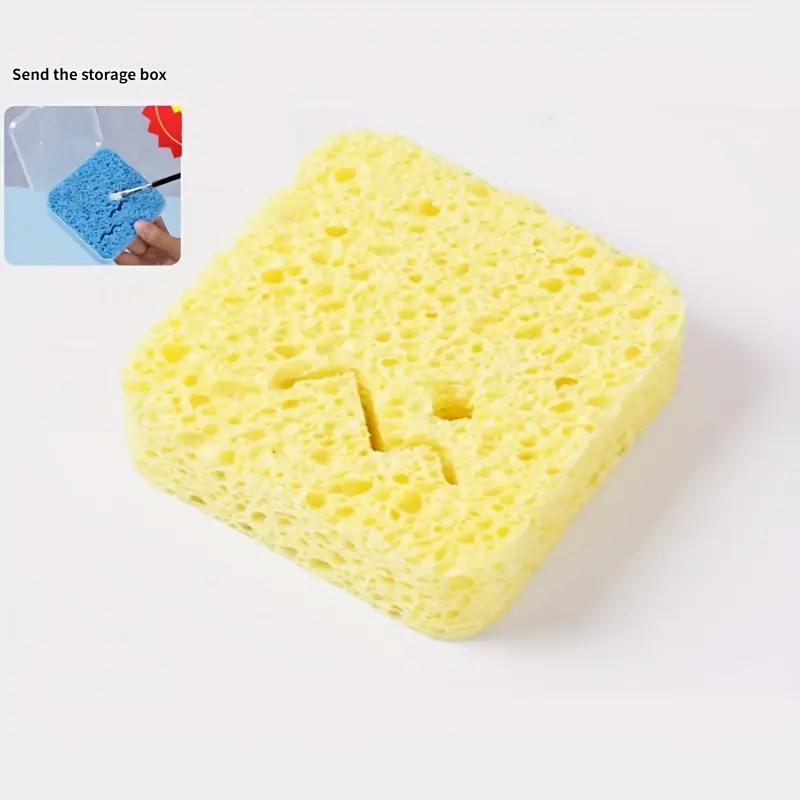The image prominently features a close-up of a yellow, square-shaped sponge with rounded edges, positioned on a plain, light gray or white background. The sponge, notable for its typical porous texture, appears to have a distinctive crack or slice resembling a lightning bolt running through its center, indicating it's starting to break. A subtle drop shadow to the right suggests the light source is coming from the upper left. 

In the upper left corner of the main image, there is a smaller, inset photograph showing a similar blue sponge inside a translucent plastic box. This smaller image includes someone's hand holding the box and a brush, possibly being used to wet the brush. Above this inset, in small black text, the phrase "send the storage box" is visible. Additionally, a partial red geometric shape is cropped into the upper right corner of the smaller image. 

Overall, the main and inset images combined provide a detailed view emphasizing the sponge's characteristics and the appearance of a storage solution.